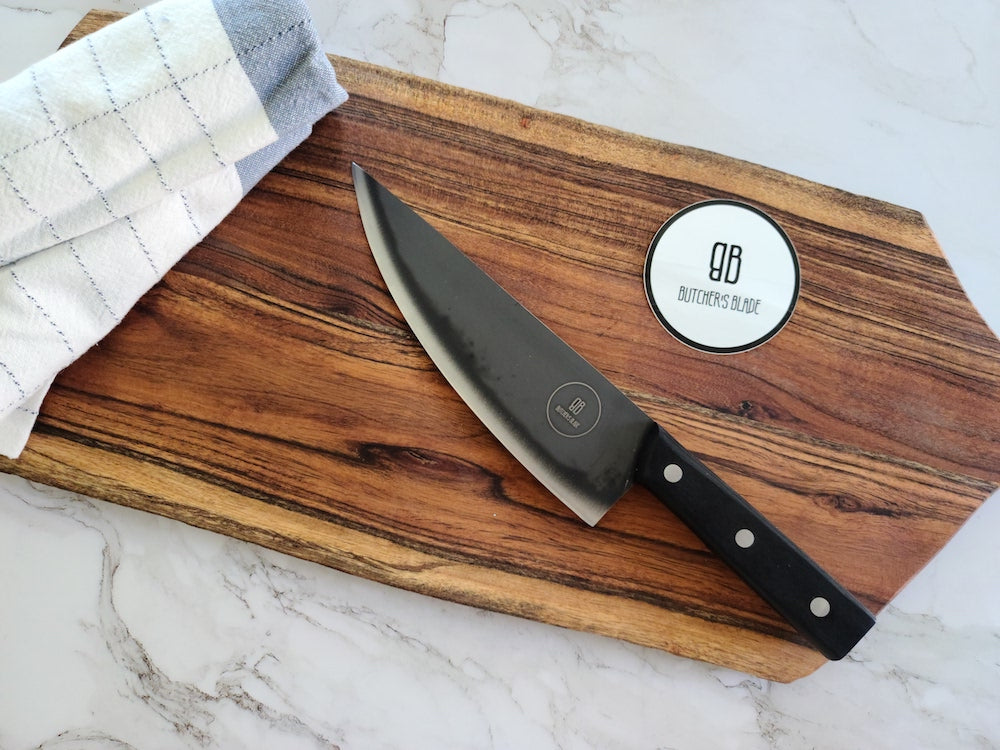The image showcases a detailed advertisement for a Butcher's Blade knife set against a pristine white and gray marbled granite countertop. Centered prominently is a natural wood cutting board, displaying rich grained patterns in tan and darker brown hues. A gray and white checkered dish towel is folded and placed on the upper left side of the cutting board. Dominating the center, a sleek chef's knife with a black handle and a sharp, stainless steel blade lies perfectly positioned. The handle features visible tail rivets adding to its robust appearance. In the upper right corner of the cutting board, a white circular sticker displays a black double "B" symbol, with the letters facing outward, and beneath it, the text "Butcher's Blade" in black. The meticulous placement and vivid details of the knife and its surroundings accentuate the high-quality craftsmanship and presentation of the Butcher's Blade.